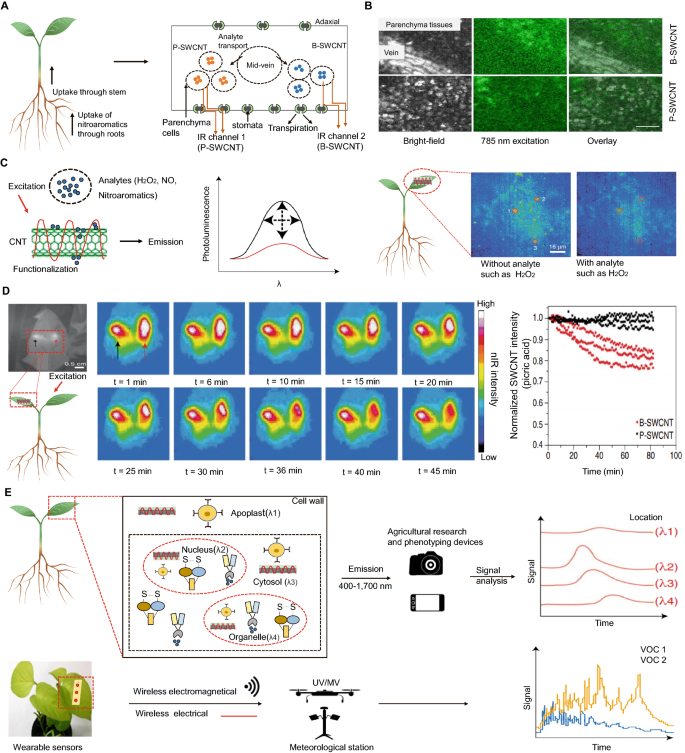The image is a comprehensive visual representation of plant growth and nutrient uptake, depicted through a series of labeled diagrams, charts, and photos, categorized from A to E. 

Label A illustrates a plant's physiological process, showcasing a stem with two leaves and visible roots. This section emphasizes the uptake of nitroaromatics through roots and stem, as denoted by arrows pointing upwards. It also includes a detailed diagram explaining analyte transport, featuring a rectangle with a mid-veined circle and smaller blue and orange dots indicating stomata, transpiration, and parenchyma cells.

Label B presents different imaging samples of plant cells, including brightfield, 785 nm excitation, and overlay images, providing varied perspectives on cellular structures.

Label C contains another explanatory chart and an accompanying photo.

Label D features multiple photos with a blue background (at least ten in total) and includes a line chart on the right side, further illustrating the data.

This detailed compilation offers an intricate overview of plant growth processes, cellular imaging, and nutrient transport systems.